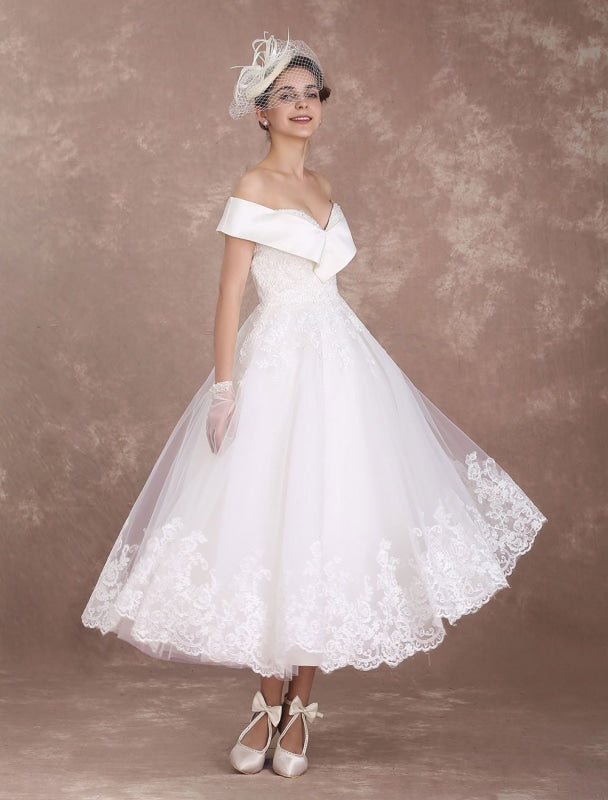In a vintage-inspired photo studio with a light cloudy gray background, a young woman poses gracefully in a 1950s-style T-length white wedding gown that stops just above her ankles. The gown features an off-the-shoulder design and a sheer outer layer edged with lace both on the hem and the bodice. The wide band of fabric elegantly frames her shoulders. She accessorizes with white knit sheer gloves edged in lace, and white satin heels with ankle straps that form a bow in the front, covering just the tops of her toes. Her hair, dark and pulled back, is adorned with a small hat embellished with a mesh veil and long, skinny feathers, positioned jauntily to the side of her head. She completes her ensemble with delicate pearl earrings in her right ear and a radiant smile, adding to the timeless charm of the photograph.